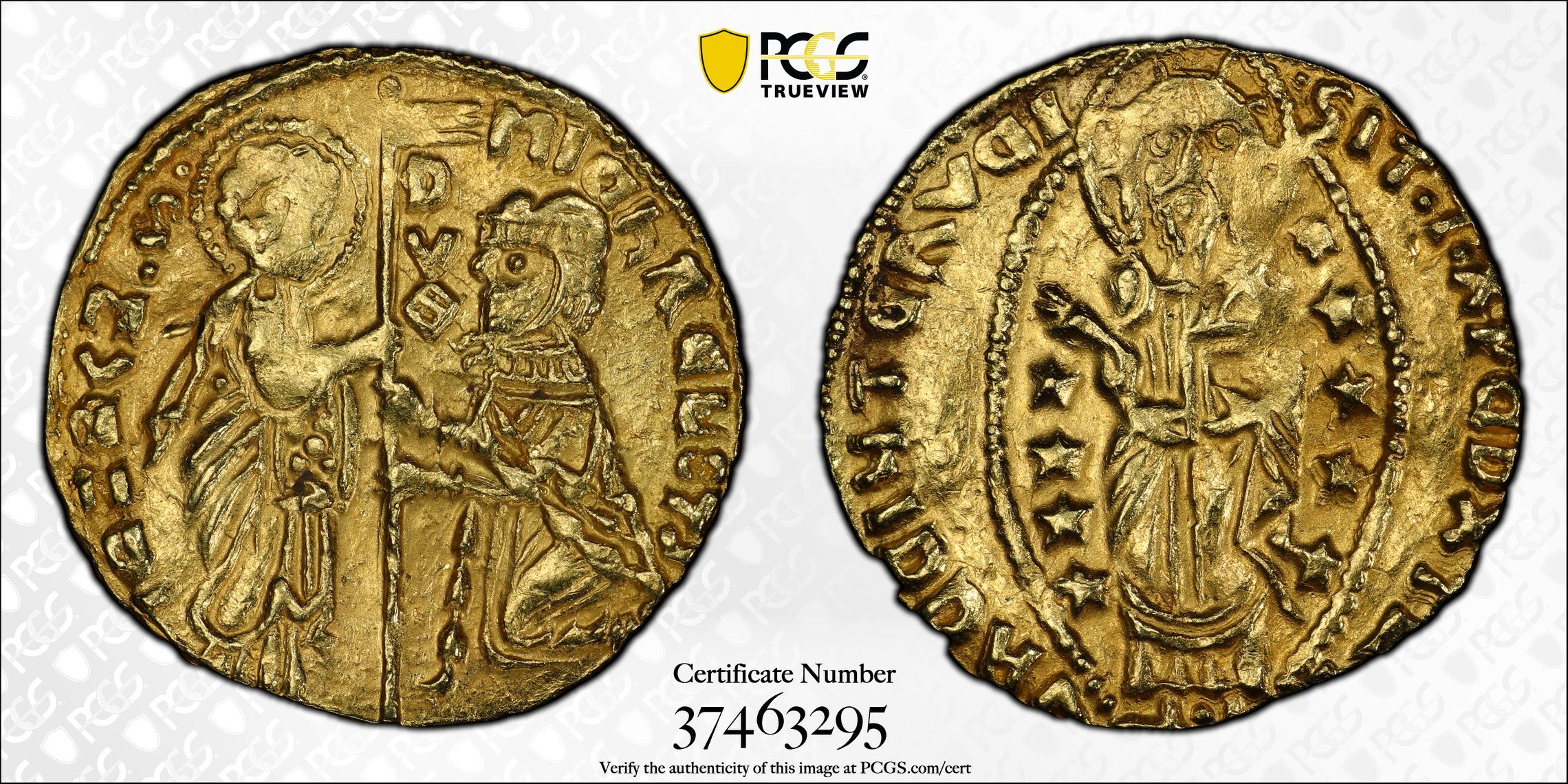This image features two ancient-looking gold coins set against a white background, accompanied by certification details from PCGS. The top of the image displays the PCGS TrueView logo, with "P," "C," and "S" in black, "G" in gold, and a gold shield emblem to the side. The bottom of the image includes the certificate number 37463295 and instructions to verify the authenticity of the image at pcgs.com/cert.

The left coin is detailed with two humanoid figures in intricate, possibly religious attire. One figure, potentially a priest or a man in a toga, holds a staff, while the other, who appears to be a knight or a Roman soldier wearing a helmet, kneels and grasps the same staff. The designs feature a variety of textures and shades of gold, adding to the ancient and tarnished look of the coins.

The right coin, though more faded and difficult to decipher, seems to include a Christ-like figure among its imagery, implying religious iconography. Surrounding both coins are illegible writings and star patterns, each contributing to the historical and intricate appearance of the objects. The coins exhibit varying textures with raised bumps and detailed engravings, evidence of their antiquity and craftsmanship.